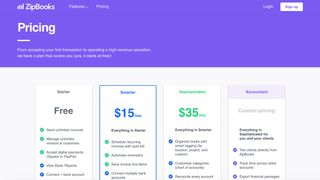This is an incredibly blurry image featuring a website page with a dark purple header. In the upper-left corner, the text "Zip Books" is faintly visible, and beside it are the words "Featured" and "Pricing," though they are somewhat unclear. On the far right side of the header, there is a "Login" option, accompanied by a white rectangular button labeled "Sign Up." Below the header, the word "Pricing" is clearly marked with a line under it, followed by an illegible sentence. 

Further down, there appears to be a section listing different pricing plans. At the top, there is a word that cannot be clearly discerned, but beneath it, the word "Free" is evident. This section contains three green boxes on the left side, followed by two blue boxes at the bottom.

Next to this, another pricing plan is displayed, labeled "$15," which also contains three green boxes and one blue box at the bottom. Further along, a "$35" plan is featured, displaying three blue boxes. On the far right, there is another pricing option without a specified price, consisting of three purple boxes.

Despite the blurriness, the image attempts to outline various service tiers provided by Zip Books, with specific features highlighted in colored boxes for each pricing plan.